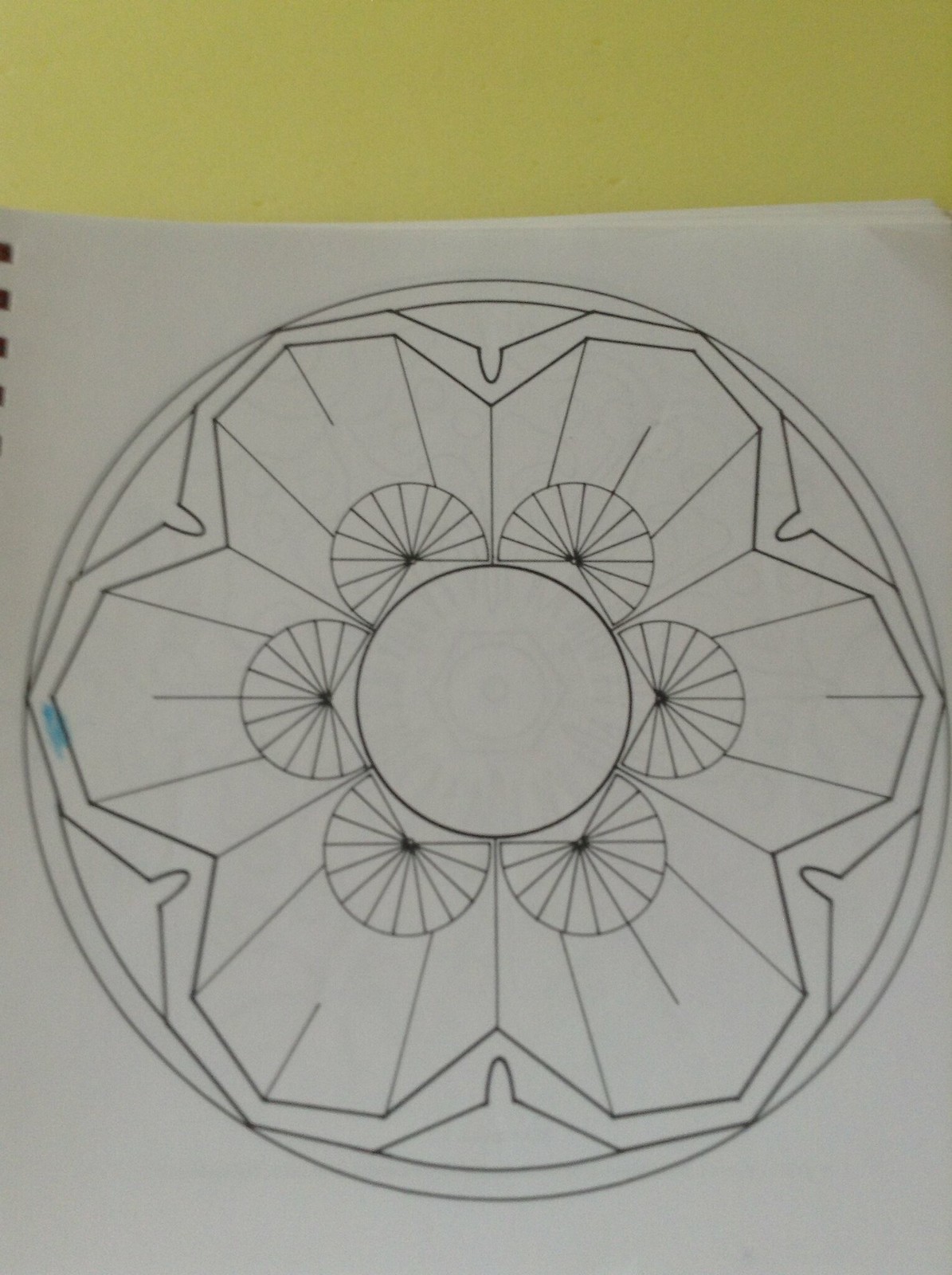The image showcases a detailed black ink drawing on a piece of white sketch paper, prominently mounted on a yellow background. The page is part of a spiral notebook, evident from the visible pages underneath and the characteristic holes on the upper left-hand corner. The central element of the drawing is a complex, symmetrical floral design. At the core, there's a central circle surrounded by smaller half-circles, each containing a black dot and radiating lines that converge at the center. This central motif resembles flower petals with intricate lines extending outward. Around this central pattern, six larger petal-like shapes form a second, expansive circle, integrated with zigzag lines and blue crayon shading that adds a touch of color on the left side. The entire design is meticulous, with layers of circular patterns, giving the appearance of overlapping petals within a grand, encompassing circle, creating the impression of a large, intricate flower.